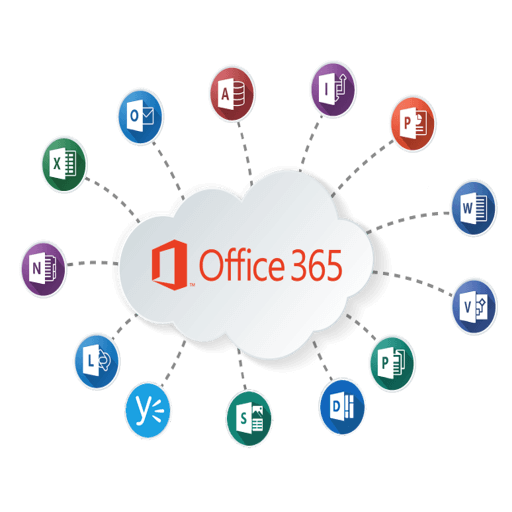This image is an advertisement for Microsoft Office 365, presented in a vibrant and engaging style. Central to the design is a prominent white cloud, symbolizing cloud-based services. At the heart of this cloud, the text "Office 365" is displayed in a bold orange font, capturing attention immediately. Adjacent to the text on the left side, there is an orange, cube-like box with a hollow center and visible walls, representing the suite of services Office 365 provides.

Extending from the edges of the cloud are dotted lines, each leading to various application icons included within the Office 365 suite. These lines illustrate the connectivity and integration of Microsoft’s services. Among these applications:
- Microsoft Excel is represented by a green icon with a recognizable "X."
- Microsoft Outlook features a blue icon with an envelope symbol.
- Microsoft Access is marked by an orange-reddish icon with an "A."
- A purple icon with an eye symbol is present, though its specific application could not be identified.
- Microsoft PowerPoint is denoted by an orange icon with a "P."
- Microsoft Word stands out with a blue icon featuring a "W."
- Microsoft Visio is also represented by a blue icon, in line with its design identity.
- There's an icon resembling Yelp, marked by blue, indicating its inclusion.
- A green icon with an "S" suggests another application, likely Microsoft Sheets.
 
Additionally, there are other icons, including a "D," "N," and "L," indicating more included applications, though their specific programs are not identified. This visually rich advertisement clearly conveys the diverse and comprehensive suite of applications offered by Office 365, making use of vibrant colors and familiar symbols to communicate the range of tools available to users.